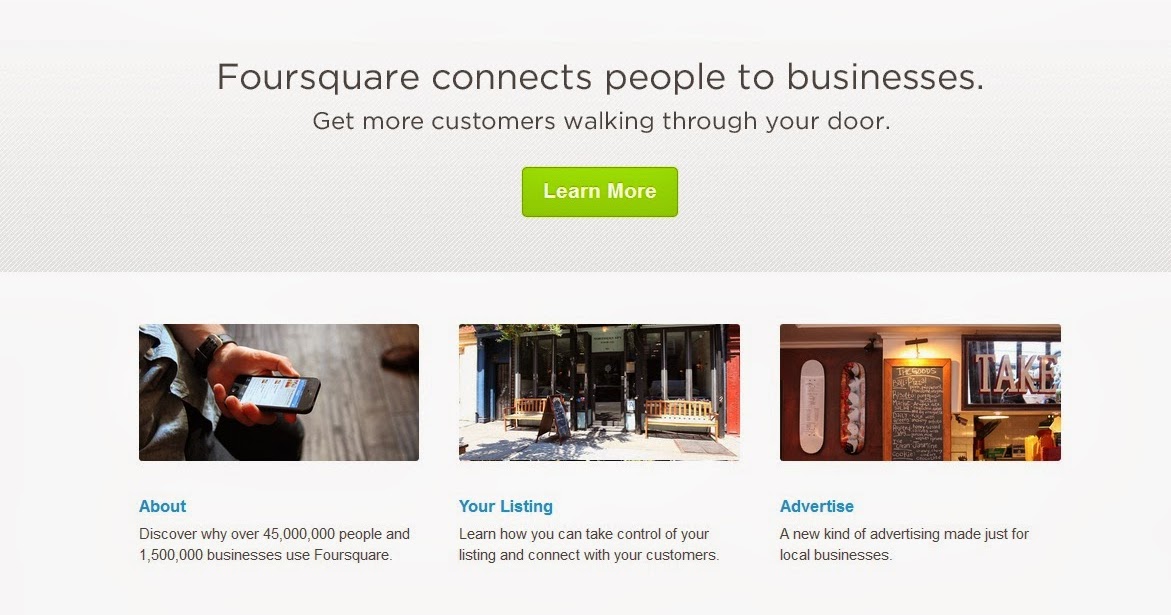The image prominently features a top half with a dark gray bezel showcasing black text that reads, "Foursquare connects people to business." In a smaller black font underneath, it states, "Get more customers walking through your door." A green clickable button with white text in the center says "Learn More."

Below that, multiple images are displayed, with the central one showing a person's hand holding a small cell phone. The person is wearing a watch with a brown strap, and the background features a brown floor. Beneath this image, blue text reads, "About," followed by black text stating, "Discover why 45 million people and 1.5 million businesses use Foursquare."

Another image depicts people standing outside a storefront with brown benches and lots on the right side, captured during the day. Below this, blue hypertext reads, "Your Listings," with additional black text encouraging users to "Learn how you can take control of your listing and connect with your customers."

The final section shows the interior of a building with a wooden door featuring oval windows. To the right, there's a window, and beneath it, the blue hypertext reads, "Advertise." In black text, it states, "A new kind of advertising made just for local businesses."